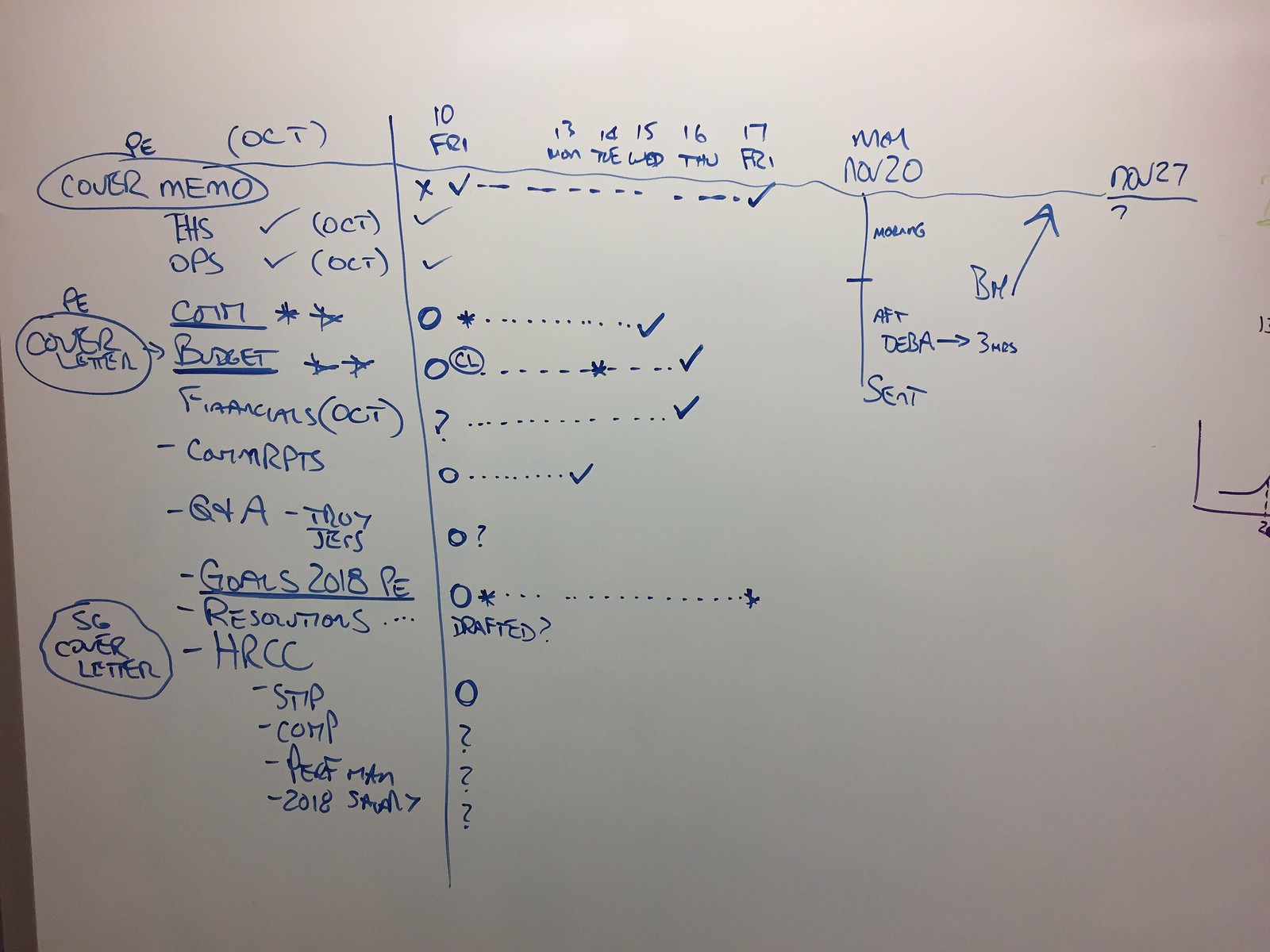This photograph captures a detailed whiteboard used for planning, possibly a class or project. The board mainly employs blue marker and displays a structured timeline at the top, beginning with October 10th (Friday), followed by October 13th (Monday), October 14th (Tuesday), October 15th (Wednesday), October 16th (Thursday), and October 17th (Friday), before jumping to November 20th (Monday) and November 27th. The content is organized into several headings and sections, starting with “cover memo,” “cover letter,” “budget,” and “financials,” each marked with checkmarks, question marks, or other indicators to show progress.

Key elements include various abbreviations such as EHS, OPS, COMM, RPTS, Q&A, HRCC, STIP, COMP, PSEF, and PE, reflecting different tasks or departments involved. Goals for 2018 are also mentioned, alongside a specific reference to a smaller column indicating “May 2020, morning, DEBA, three hours, and seat,” and an uncertain date, “NOV27,” denoted with a question mark. These notes suggest a timeline of events, anticipated actions, or milestones. The board's central section features these dates and goals, highlighted with diverse symbols like X's, checks, dashes, and dots, though their exact meanings are not provided. The overall scene suggests meticulous planning with ongoing updates, highlighted by an absence of clarity on the full context or the intended outcome.